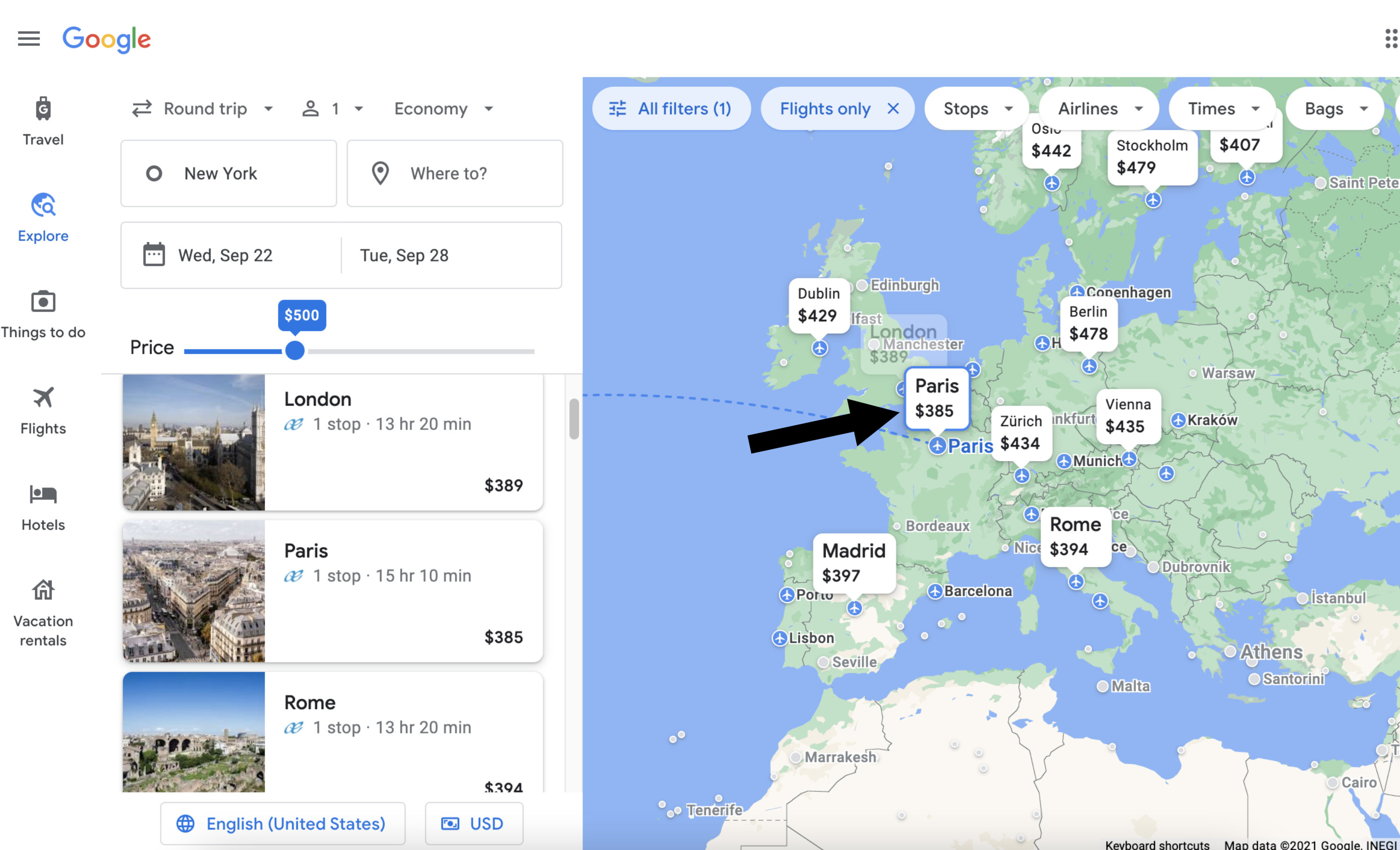A Google search results page displays a map of Europe focused on travel plans, indicating searches related to flights. The map prominently shows destinations like London, Paris, Manchester, and Rome. Speech bubbles above these cities display flight prices: $385 for Paris and $389 for London. Travel dates are specified as Wednesday, September 22nd to Tuesday, September 28th. An arrow highlights the Paris speech bubble, with London's information faintly visible below it. Various filter options are available on the map, including "Flights only," "Stops," "Airlines," "Times," and "Bags." The map bears a 2021 copyright notice.